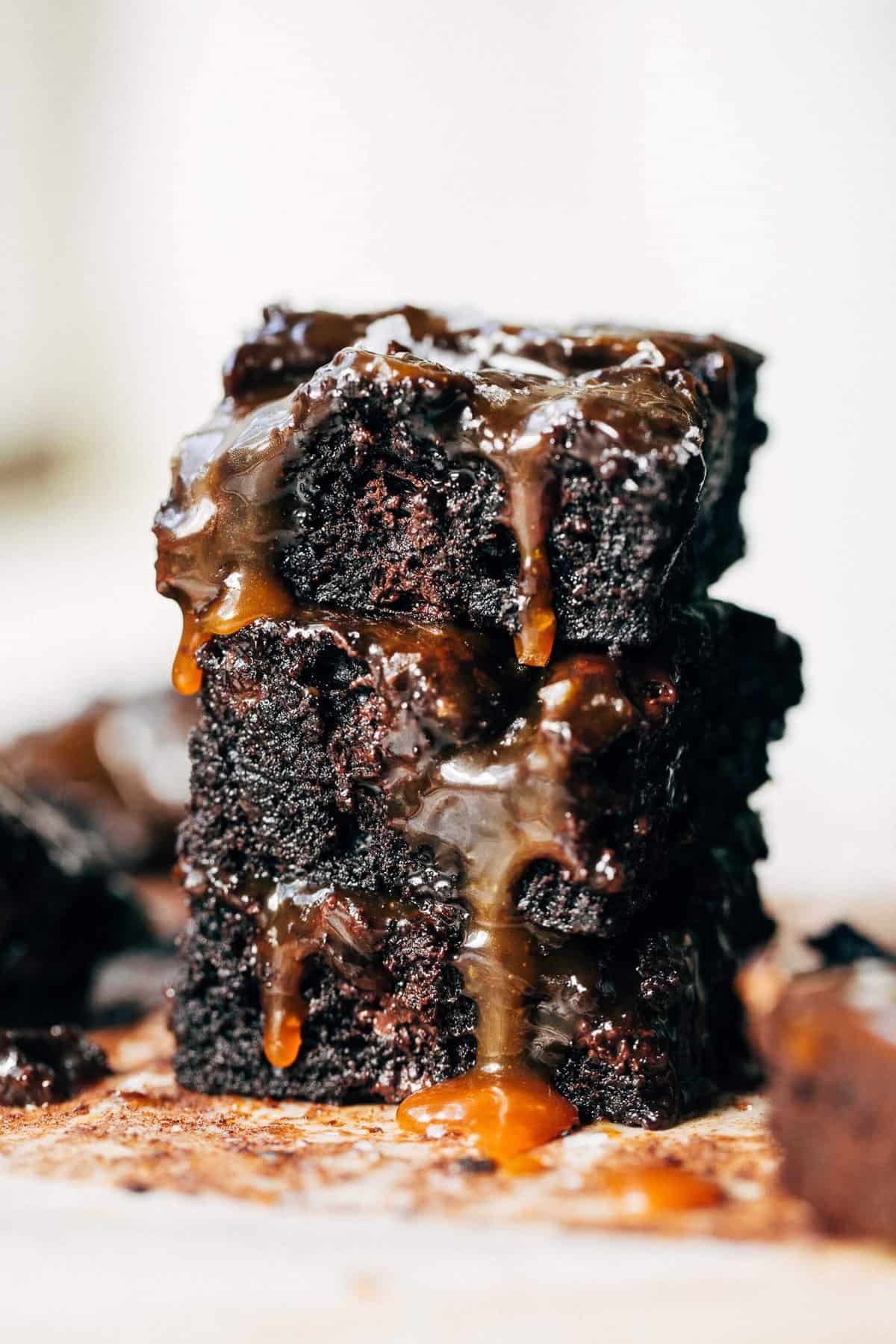The image depicts a vertical rectangular photograph with a blurred gray background, emphasizing the main subject—a tantalizing stack of three dark, moist brownies. These decadent brownies are generously drizzled with a rich caramel sauce that cascades over the edges, pooling slightly around the base. The brownies are arranged with two larger pieces on the bottom and a slightly smaller piece on top, creating a visually appealing layered effect. The stack rests on a brown surface that might be parchment paper, with traces of brownies and caramel indicating where they adhered. Additional pieces of brownies are visible in the background, and stray dribbles of caramel sauce add to the indulgence. On the left side, another partial brownie can be seen, enhancing the depth of the image.